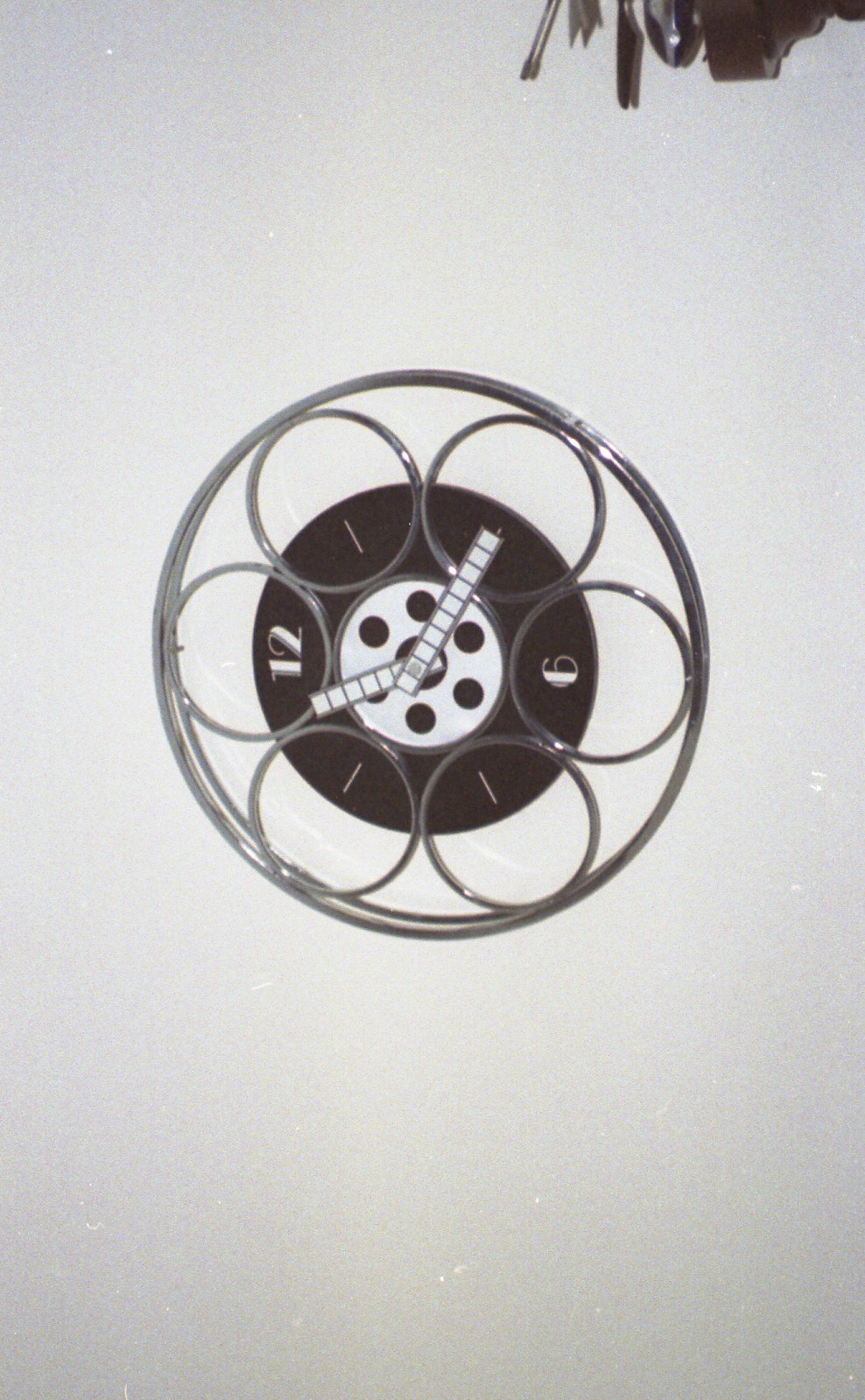The image features a uniquely designed clock, hanging on a white wall. Unlike traditional clocks, this one is positioned on its side, with the numbers 12 and 6 aligned horizontally. The clock face is intricate, resembling a film reel or perhaps the barrel of a gun, with a large central circle enveloped by smaller circles, all rendered in white.

The clock's minute and hour hands are boldly styled, resembling a grid of white blocks outlined in silver or chrome. Surrounding the central motif is a pattern that evokes the appearance of interconnected chrome rings, forming a flower-like design.

Encasing this elaborate arrangement is a larger chrome ring, adding to the clock's striking and unconventional appearance. The image captures the clock against a white wall, with the bottom edge of a shelf just visible at the top of the photo.